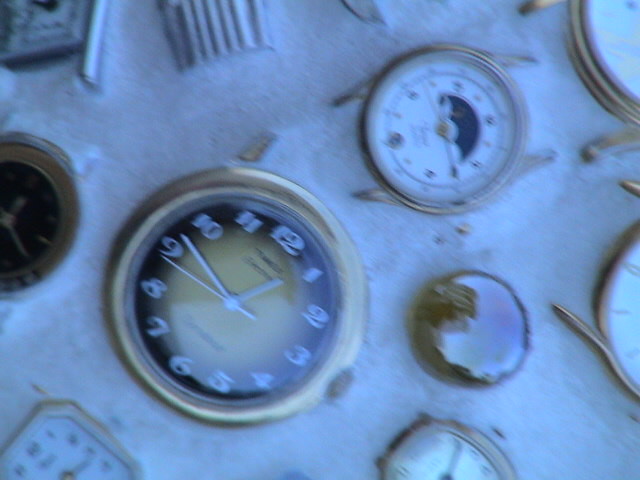The photograph captures a slightly out-of-focus collection of various watch faces scattered on a light-colored, beige-dotted surface, possibly a white cloth in a watch repair shop or jeweler's workspace. Dominating the center of the image, there are two round watch faces: one features a gold-colored rim with a matching gold face, accented with a black border and Arabic numerals, complementing the silver or white watch hands, including a second hand. The other central watch face is white encased in a gold circle, displaying a distinctive blue umbrella shape. Around the edges of the image, numerous other watch faces—mostly round with one appearing octagonal—are partially visible, contributing to the clutter of the scene. Notably, at the top left is a black watch face with a gold border, while the bottom left corner reveals what seems to be a square white watch face. Additionally, a white compass with blue markings is discernible at the top right, adding to the assortment of timepieces and perhaps hinting at the tools or parts used for watch repair evident in the scene.